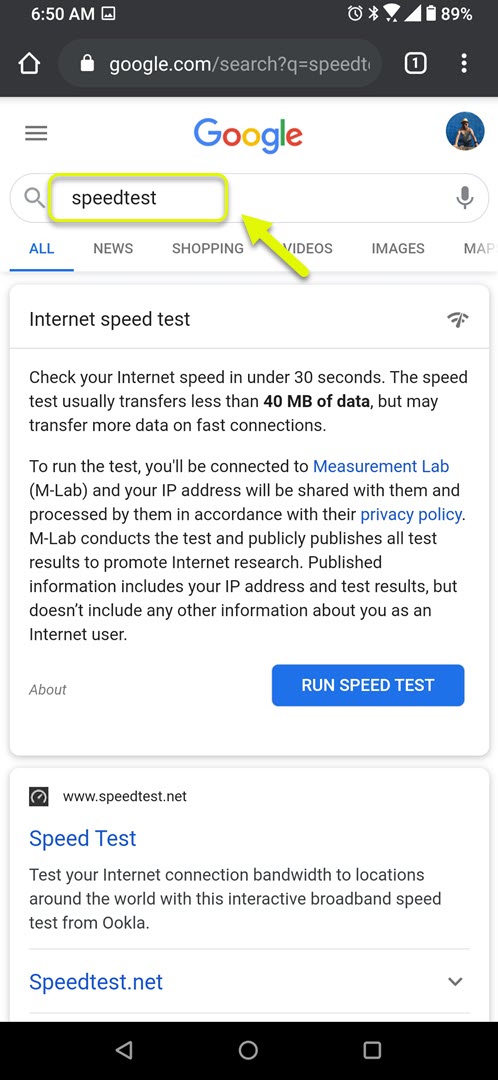Certainly! Here’s a cleaned-up and detailed caption for the image described:

---

In the image, a smartphone screen displays a black status bar at the top with white indicators showing the time "6:50 AM" on the top left. To the right, icons indicate the clock, a pie-shaped symbol representing Wi-Fi connectivity, and a battery icon showing "89%."

Mid-screen, on the bottom right, there's a view of the Google search page, including a white padlock symbol next to "google.com" indicating a secure connection. The search URL shows "google.com/search?q=speed" in grey text, with a white square containing the number "1" and three dots.

The Google logo is prominently centered, displaying the letters "G" in blue, "o" in red, "o" in yellow, "g" in blue, "l" in green, and "e" in red. To the right of the search bar is a grey microphone icon. Below the search bar, there are blue underlined text options: "News," "Shopping," "Videos," "Images," and "Maps."

Further down, a section titled "Internet speed test" includes a Wi-Fi logo on the right. The text below reads: "Check your internet speed in under 30 seconds. A speed test usually transfers less than 40 MB of data, but may transfer more on fast connections. To run the test, you'll be connected to Measurement Lab (M-Lab) and your IP address will be shared with them and processed by them in accordance with their privacy policy. M-Lab conducts the test and publicly publishes all test results to promote internet research. Published information includes your IP address and test results, but does not include any other information about you as an internet user."

Below this, in grey text, it reads "About." Further below, a blue button labeled "Run Speed Test" in white text is visible. Underneath, a section displays "www.speedtest.net" with the title "Speedtest" in blue. The accompanying text says, "Test your internet connection bandwidth to locations around the world with this interactive broadband speed test from Ookla." 

A grey line is followed by "speedtest.net" in blue text with a grey arrow pointing to the right. Towards the bottom, a black box with a grey triangle pointing left, a white rounded circle in the middle, and a white square to the right completes the image.